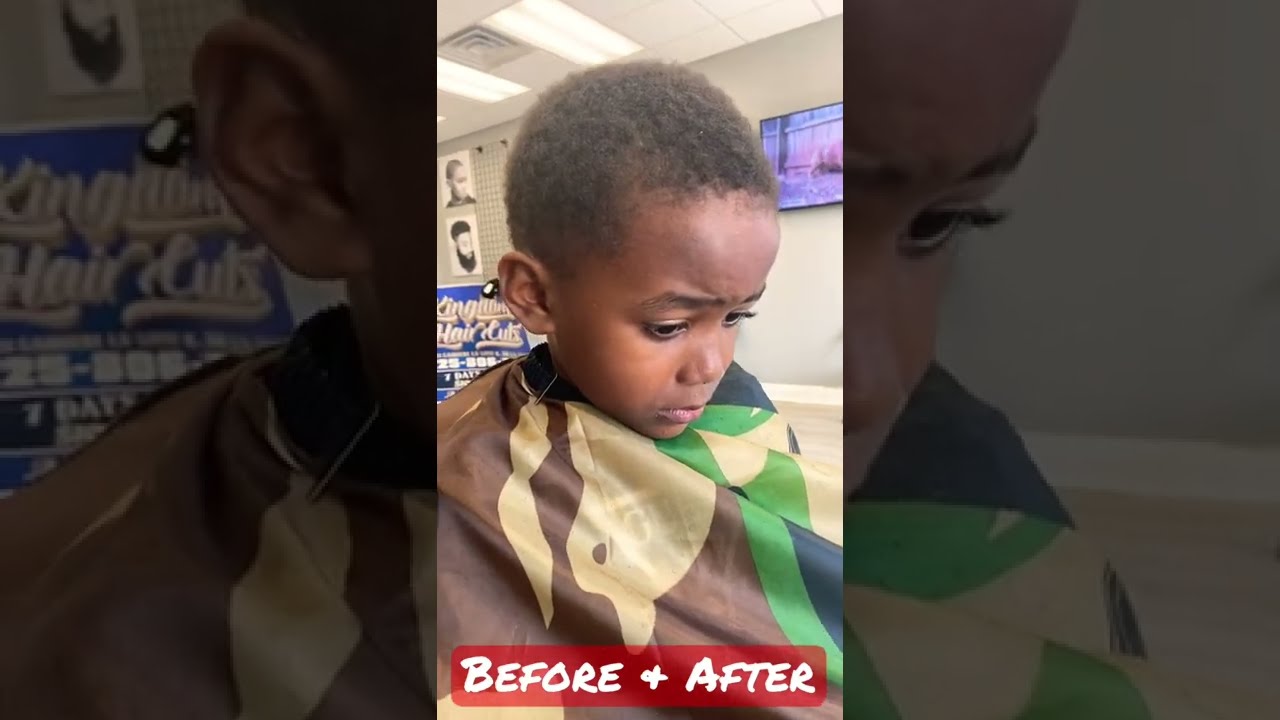In the center of this image, there is a small black boy, approximately 5 or 6 years old, sitting in a barber shop chair. He appears sad or nervous, looking down toward the ground with a hesitant expression. The boy is wearing a camo-colored hair cape in shades of brown, green, and tan. The photo seems to be a screen grab from a vertically oriented cell phone video. 

The background reveals a brightly lit barber shop with a drop ceiling featuring fluorescent lights. On the wall behind the boy is a television screen, and to the left, there are pictures showcasing different men's haircuts as well as a sign indicating “Kingdom Haircuts - Seven Days.” The bottom of the image displays a red box with white text reading "before and after." Notably, the image is duplicated with a darker, enlarged version forming the background, contrasting the brighter main image centered in the frame.